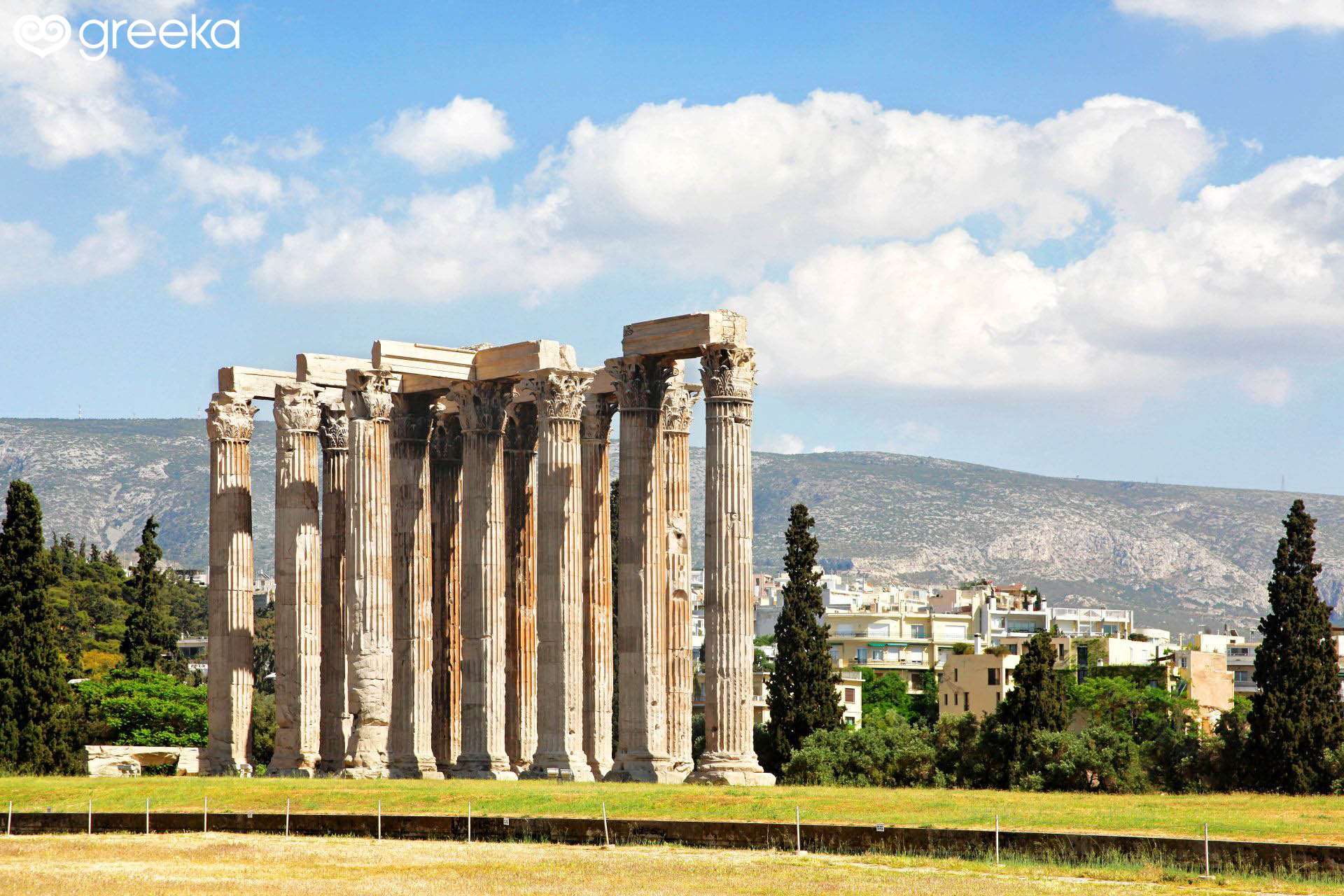This outdoor photograph captures the timeless beauty of ancient Roman columns standing together in a grassy lawn. There are precisely 13 weathered stone columns, adorned with intricate leaf pediments at their tops, arranged in a row. These ancient structures, devoid of any connecting building, evoke a sense of historical grandeur. The scene is framed by a variety of greenery, including low shrubs and towering trees. Beyond the verdant foreground, a modern cityscape with a mix of white and tan buildings stretches out, hinting at apartment or business purposes. Farther in the distance, a tree-covered mountain adds a majestic backdrop under a blue sky dotted with white clouds. The top-left corner of the image features the word "Greca," suggesting this may indeed be a snapshot from Greece, though no further identifying details are present. A subtle chain link fence runs across the front of the ruins, framing this harmonious blend of ancient and contemporary elements.